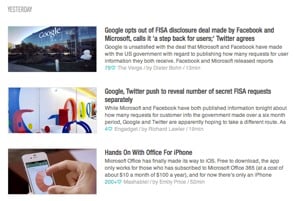The image features a completely white background. In the upper left corner, there is some underlined gray text that is too small and blurry to read. The text stretches to the far right of the image, where there is blank space. Along the right side of the image, there is an exterior shot of a glass building. The word "Google" is faintly visible in white on the building. Next to the building, there is some extremely small and dark black text, followed by several lines of lighter black text that are illegible.

Further down, there's an interior view of the Google office, displaying the colorful Google logo with the blue, red, yellow, and green letters. Beneath the logo, there is a mix of black text that includes the readable words "Google," "Twitter," and "Push," while the rest remains unreadable due to the small font size. Below this scene, a generic image of a smartphone or Android device is shown, with a white hand attempting to zoom in on the screen. Above the smartphone, there is black text that reads "Hands-on with Office for iPhone." There is additional, barely legible, small black text scattered throughout the image, which remains unreadable due to its diminutive size and the image's overall resolution.